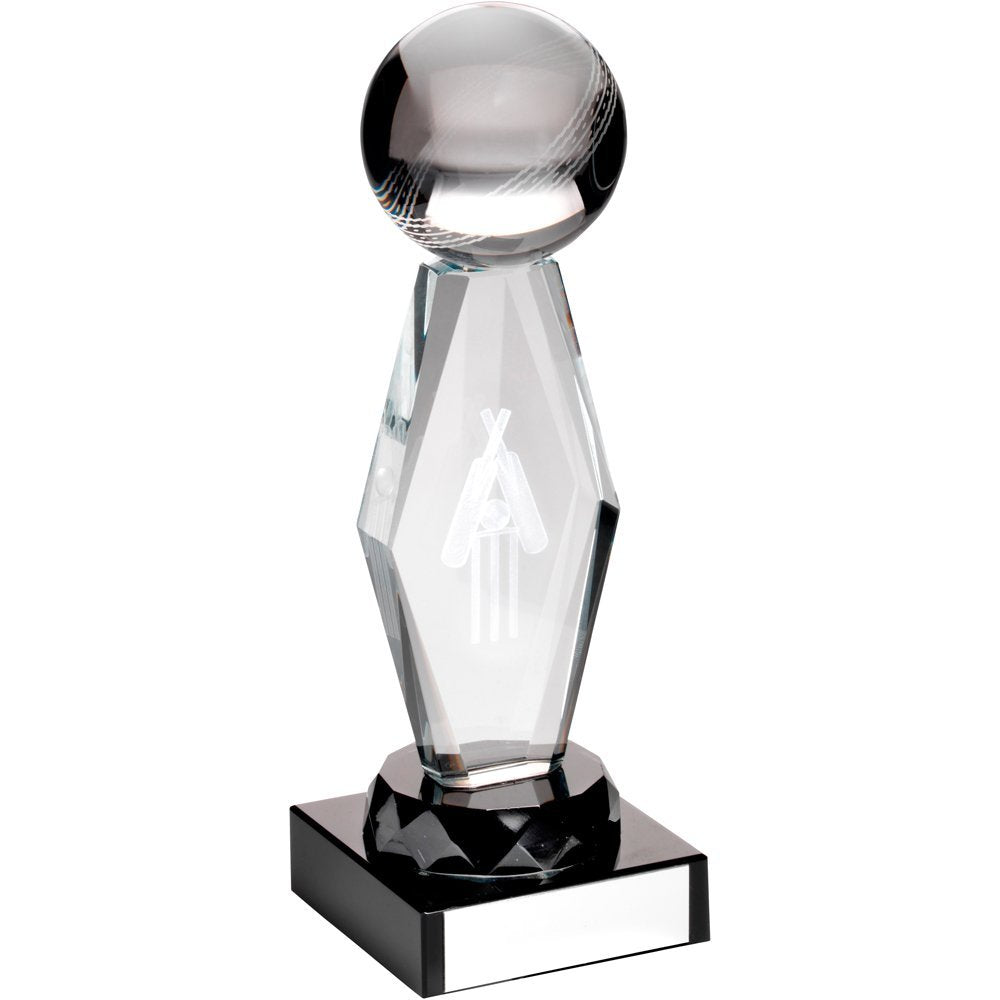Set against a white background, this elegant glass trophy features a spherical top, primarily white with some black on either side, and adorned with thin, wispy white lines encircling the sphere. The sphere rests slightly tilted at an angle. Below the sphere is a rhombus-shaped pedestal, crafted from a similar glass material. At the heart of this glass rhombus, an engraving displays two cricket bats crossed over a horizontal letter 'E', with a ball situated between the bats. The rhombus itself creates an elongated hexagonal silhouette. Supporting this intricate glass structure is a robust, black base shaped like a square, with a white plaque mounted on its front. This base forms the stable foundation of the trophy, meticulously detailed and indicative of sporting excellence.